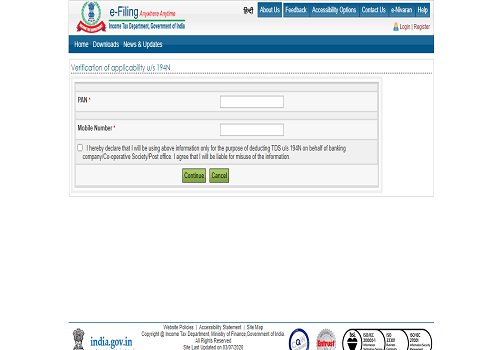The image depicts the homepage of the Income Tax Department website of the Government of India. Due to the low resolution, the text is not entirely clear, but certain elements are discernible. The background of the website is predominantly white. 

At the top left corner, the emblem of the Indian Constitution is visible, with the word "E-Filing" written next to it. Underneath, the text reads "Income Tax Department, Government of India."

To the right of these headers, a menu is shown with options such as "About Us," "Feedback," "Accessibility Options," "Contact Us," and possibly "E-Aadhaar." Further right, links labeled "Login" and "Register" can be seen.

Below this header, a blue navigation bar is present. On the left side of the blue bar, options labeled "Home," "Downloads," and "News and Updates" are visible.

In the main section of the page, set against the white background, there's a prompt that seems to involve verification of applicability, though the exact wording is unclear due to the image resolution. Below this, there are text boxes where users are expected to enter their PAN number and mobile number. There's also a declaration checkbox that users must tick, presumably to confirm that the information provided will be used solely for TDS (Tax Deducted at Source) purposes, though the complete text is not readable.

At the bottom of this section, two green buttons labeled "Continue" and "Cancel" are present.